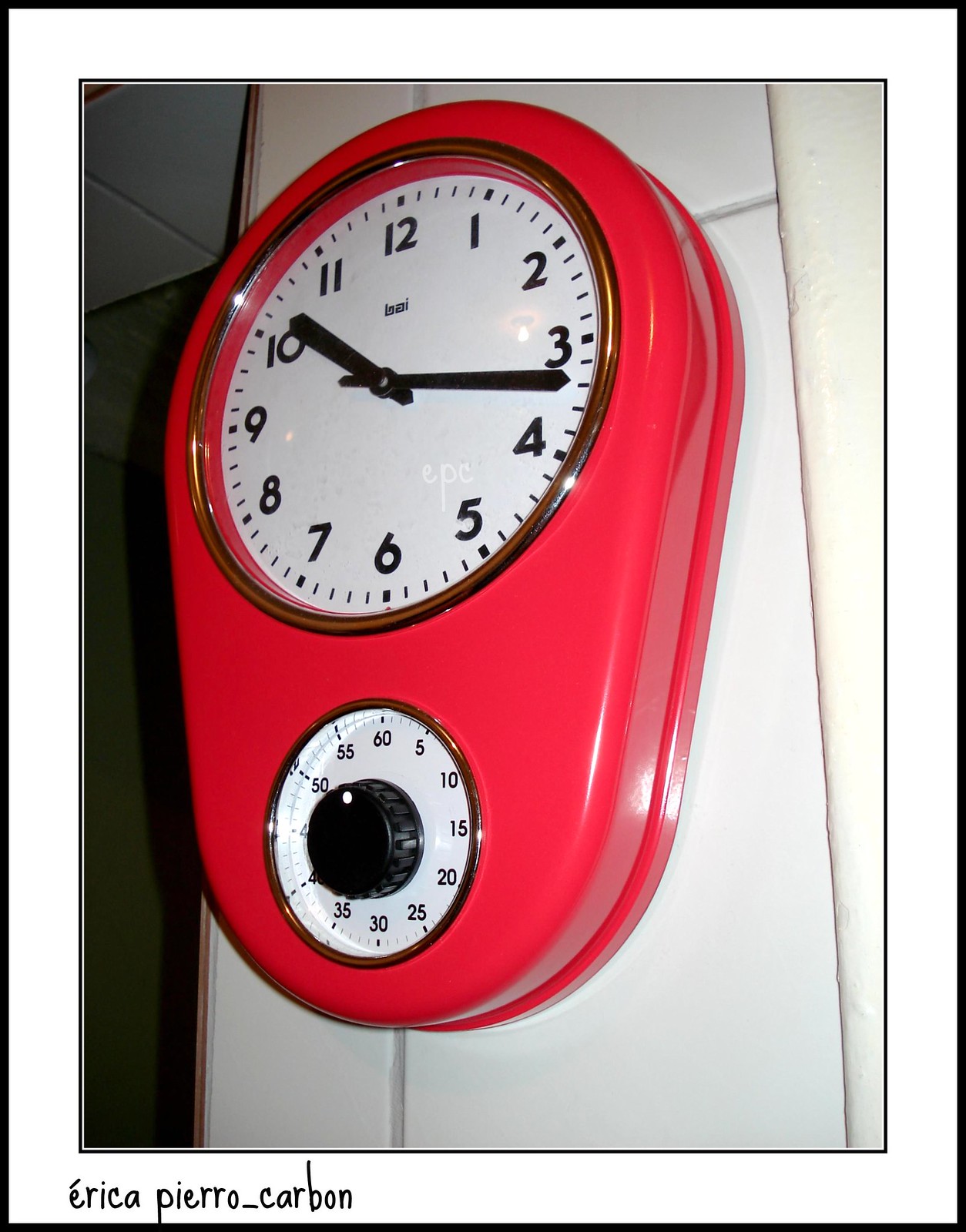The image features a unique red clock with a somewhat unconventional design. The clock has a round base and an overall rectangular shape with rounded ends, giving it an oval-like appearance. The upper half of the clock showcases a large white-faced clock dial with black numerals ranging from 1 to 12, indicating the hours. Below this, the bottom half contains a smaller white-faced circular dial, bordered by numerals in increments of 5, from 5 to 60, indicating minutes or seconds. This smaller dial is operated by a black knob located on its face. The clock is mounted on a white wall, with a white ceiling visible above. To the left of the clock, there is a shadow that suggests a hallway. The photo itself has a white border, and in the bottom left-hand corner of the border, the text "ERICA PIE RRO UNDERSCORE CARBON" is written.